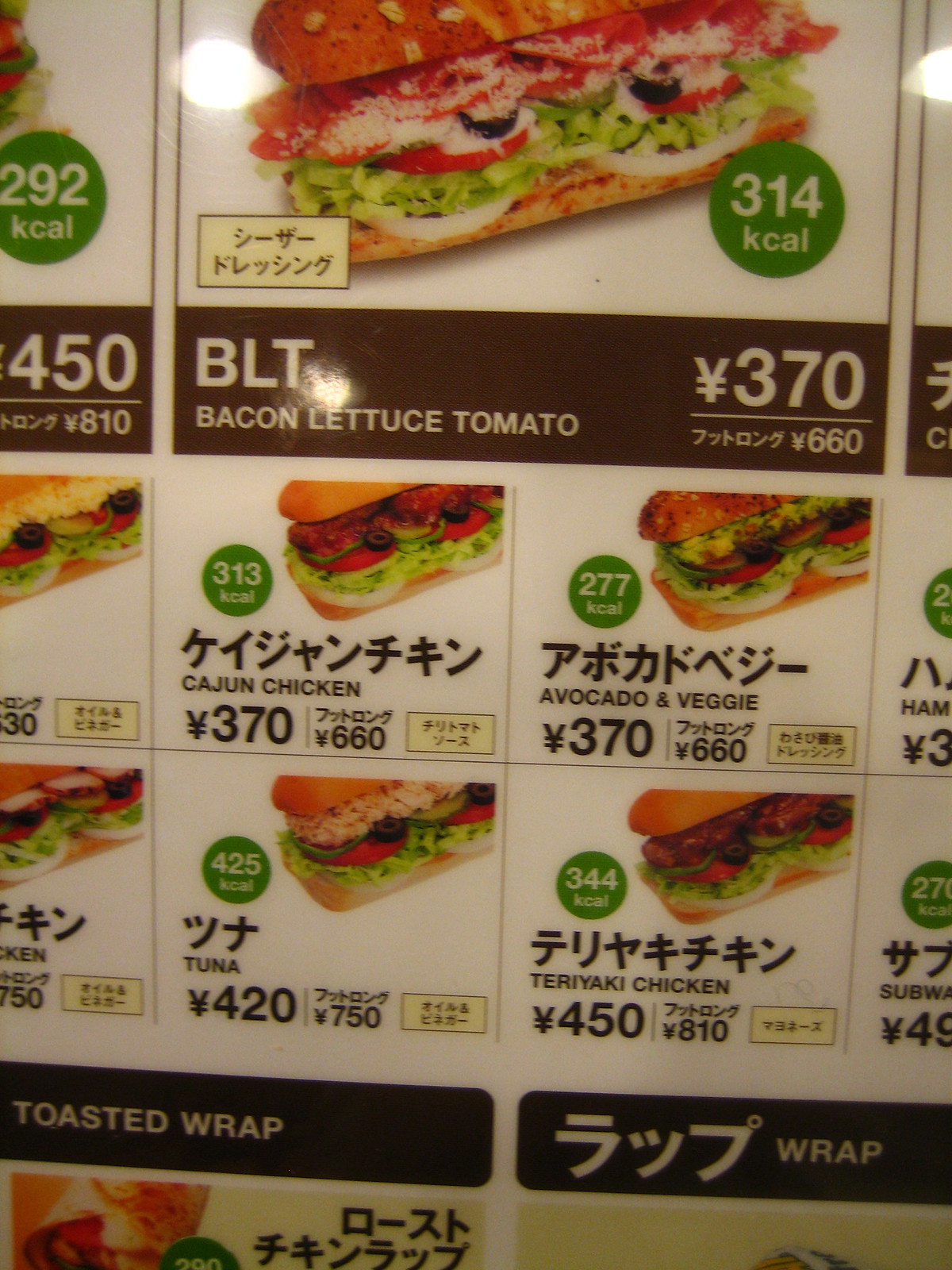This image depicts a detailed menu from a sandwich shop, organized with a clean white background accented with yellow and black text. The central part of the menu features a 2x2 grid of different sandwich options, each confined within small, distinct squares. At the top of the menu, there's a visually prominent BLT sandwich adorned with red tomatoes, lettuce, and possibly onion rings, and it is labeled with 370 yuan and 314 kilocalories. 

To the bottom left within the grid, there is a description of a Toasted Wrap and towards the bottom right, simply a text reading "Wrap". Each menu item is clearly listed with corresponding calorie information, which is displayed in small green circles with white text. Notable sandwich options include Cajun Chicken (313 kilocalories, 370 yuan), Avocado and Veggie (277 kilocalories, 370 yuan), Tuna (420 yuan), and Teriyaki Chicken (450 yuan). 

The overall layout and style of the menu suggest it is a snapshot from a sandwich shop, with a clear emphasis on nutritional information and pricing to help customers make informed choices.